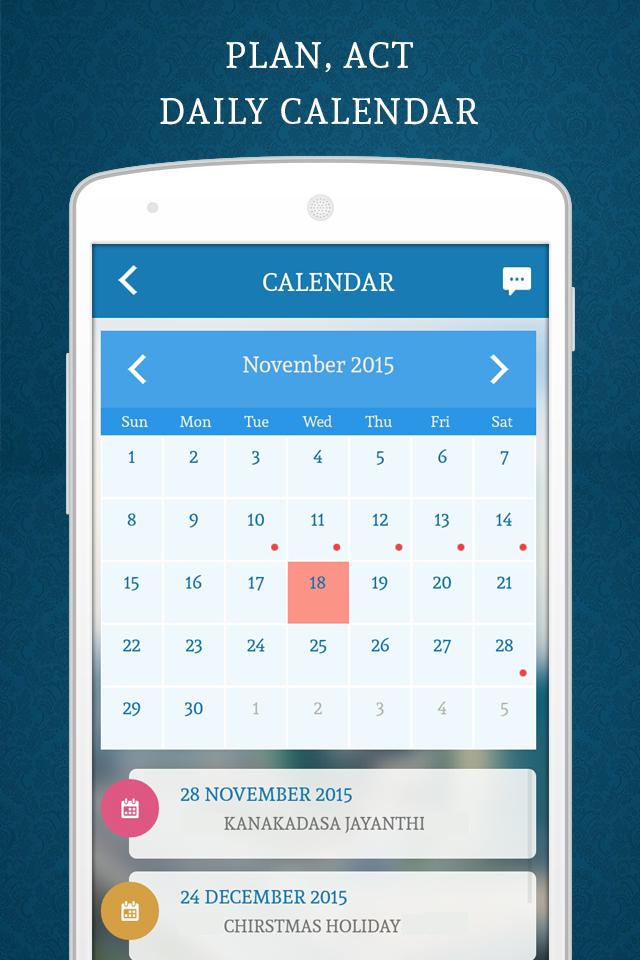The image showcases a sleek, mobile app designed for daily planning. The app's interface is set against a stylish navy blue background. At the top of the screen, bold white text prominently displays the words "Plan and Act," with the subtitle "Daily Calendar" situated just below. 

Centered in the foreground is a detailed illustration of a white mobile device. The device features volume up and down buttons on its left side and a power button on the right. The mobile device's frame and face are both white, creating a clean and minimalist look that complements the app's aesthetic.

On the device's screen, a blue and white themed calendar interface is visible. The top of the calendar screen features the word "Calendar" with a small message icon situated to the right. The date displayed is November 2015, with particular emphasis on dates 10th, 11th, 12th, 13th, 14th, and 28th, each marked with red indicators suggesting upcoming events or important dates.

Beneath the calendar grid, entries for specific events are listed for November 28th and December 24th, giving the user a quick glance at noteworthy upcoming activities. The meticulous design and user-friendly layout of this daily planner app make it an essential tool for managing one's schedule effectively.